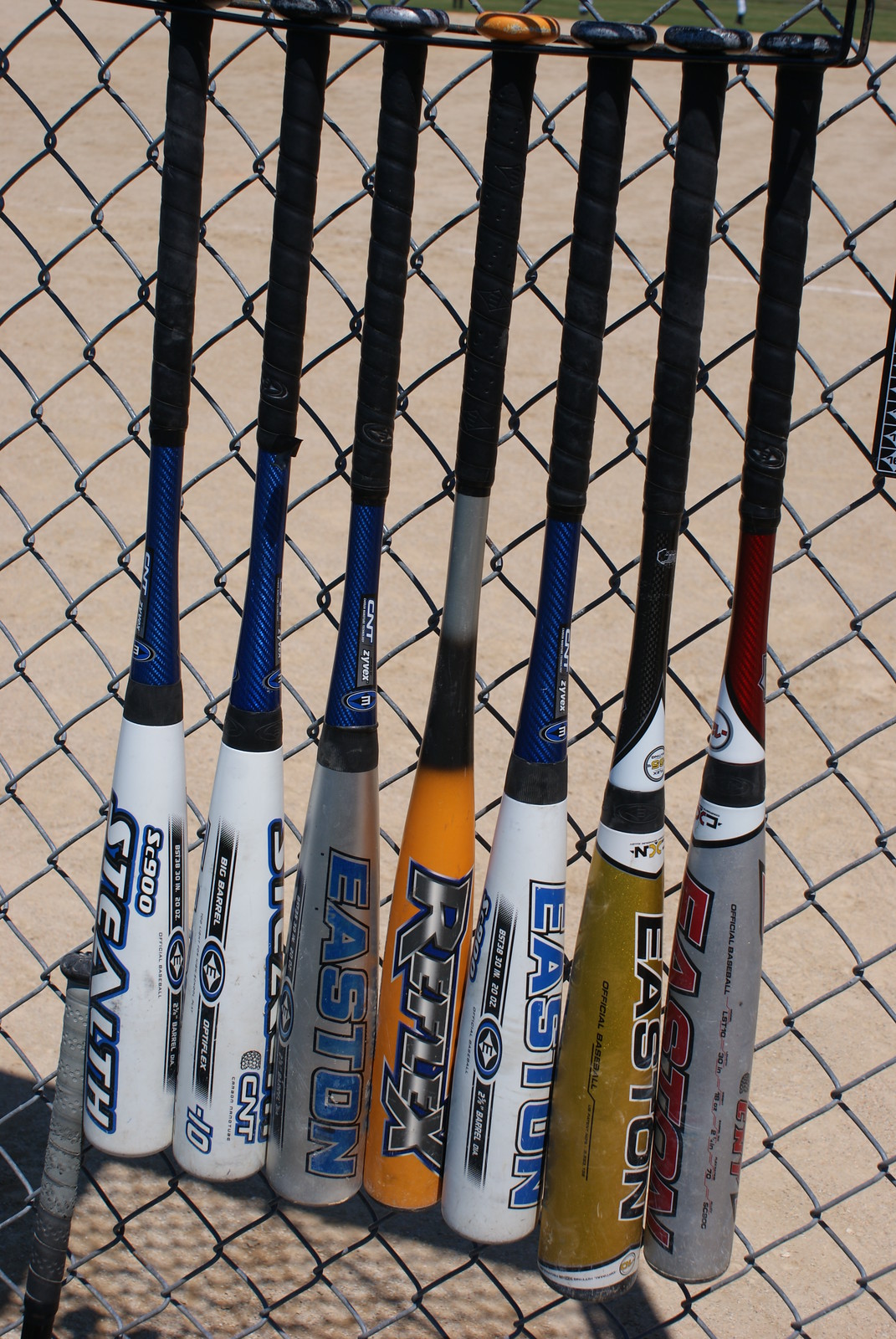This image features a collection of seven aluminum baseball bats meticulously lined up and suspended upside down by their knobs from a chain-link fence. Behind the fence, the sandy-colored ground of the baseball diamond and patches of green grass are visible. One additional bat rests on the ground, leaning against the row of hanging bats, ready for use. Each bat, predominantly made by Easton, showcases a variety of colors and model names, including "Reflex" and "Stealth." The bats display a spectrum of colors: two are white, one is silver, one orange, one is gold, another is gray with red lettering, and another is navy blue. All bats are equipped with black handles. The sunlight casts intricate shadows of the fence onto the sandy ground, adding depth and texture to the scene. The neatly organized bats signify preparedness for the upcoming baseball game.